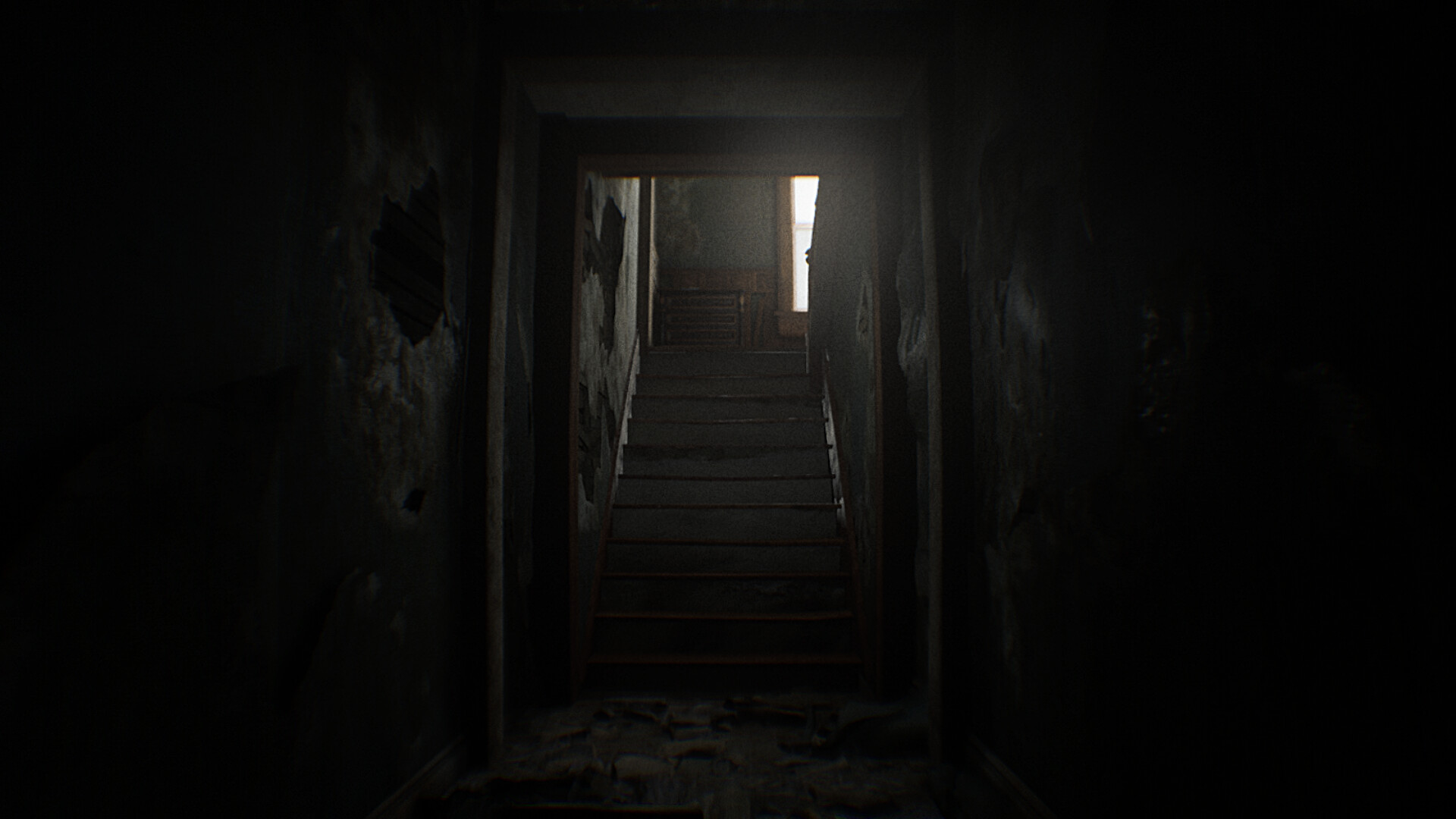The image captures a dilapidated and abandoned hallway leading to a stairwell. The perspective is from the center of the hallway, looking towards a doorway through which a staircase ascends. The wood-framed doorway sits amid walls that once had wallpaper or paint, now peeling away and contributing to the overall decay. The stair steps are a dark wooden hue, with scattered debris littering the floor at the base. Both the left and right walls are gray, riddled with holes and appearing to crumble. At the top of the stairs, a partial view of a brown, wooden-trimmed window is visible, surrounded by more gray wall and wood paneling at the bottom, reinforcing the sense of neglect and abandonment enveloping the space.